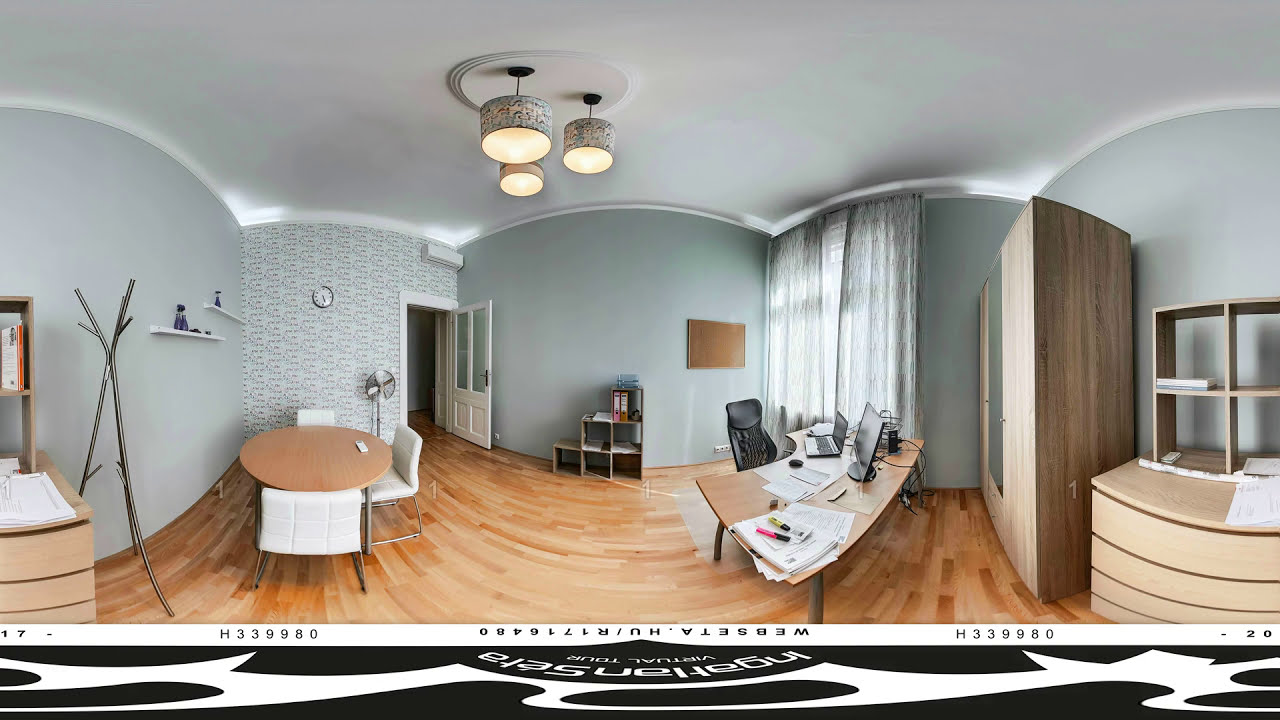The image captures a meticulously arranged modern office space, seemingly photographed for a brochure or similar promotional material. The room features a harmonious blend of grayish-blue painted walls with an accent wall adorned with wallpaper, contributing to its stylish and contemporary aesthetic. The floor is comprised of wooden slats in a lighter shade, complementing the modern wooden furniture found throughout the space.

A notable element in the lower-left quadrant of the image is a round wooden table surrounded by three white chairs, adding to the office's sleek design. To the right, a window draped with sheer curtains allows natural light to filter into the room. Prominent in the scene is a desk equipped with a black chair, a computer, monitor, and various office supplies such as papers and pens, reinforcing the room's functional yet polished look.

Additional furnishings include cube storage units, more shelving and storage options on the right, and an open white door featuring glass panels. Noteworthy is the inverted black-and-white text at the bottom of the image, likely detailing information about the photograph or the photographer, enhancing the professional presentation of the space. The overall setup, possibly captured using a 360 lens or Matterport software, ensures a comprehensive view of the office's sophisticated interior.